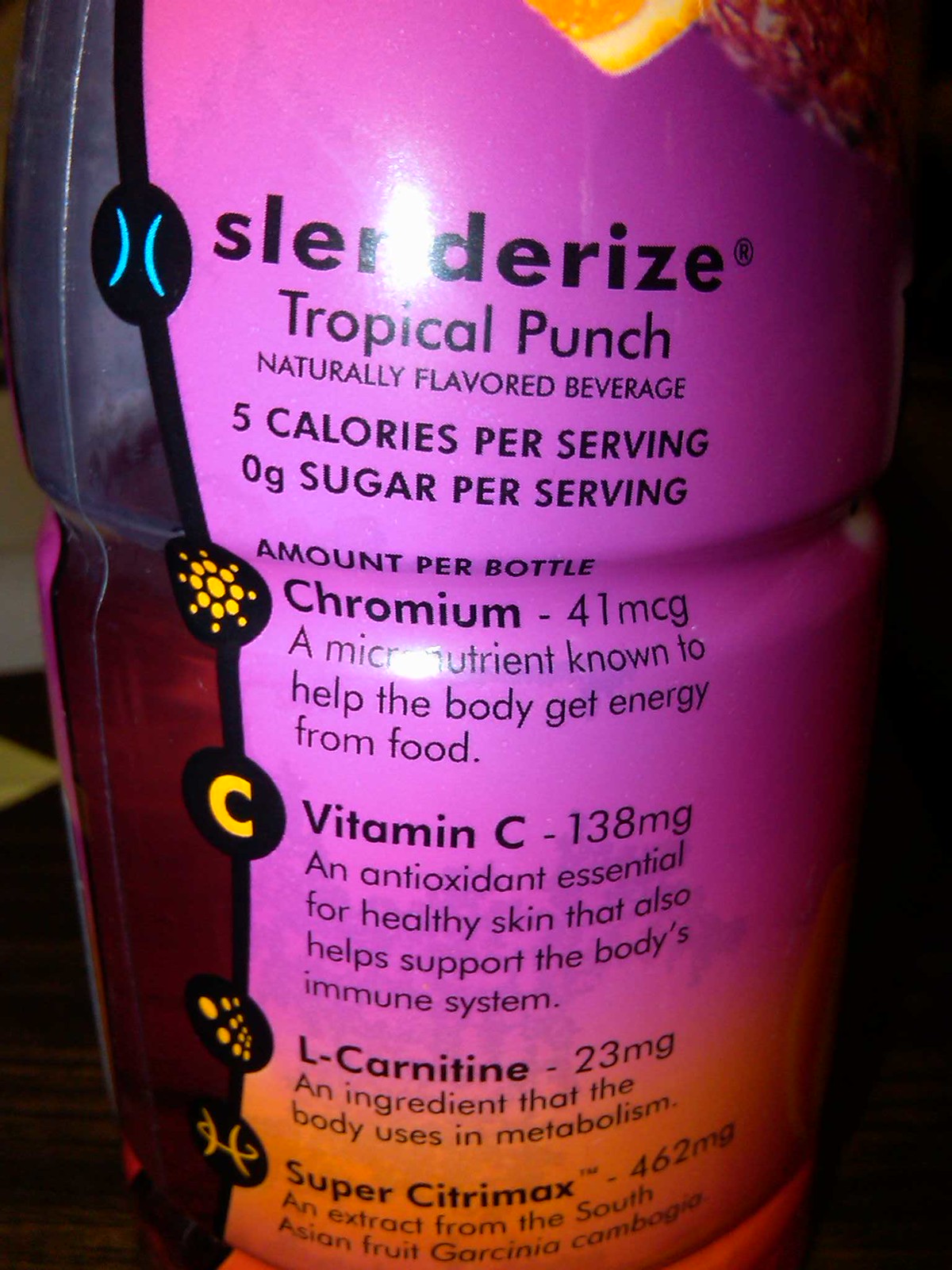The photograph features a close-up of a beverage label, specifically a “Slender Ice Tropical Punch” drink. The label is primarily purple, with sections that are clear, allowing a glimpse of the beverage inside. The main focus is on the nutritional benefits and ingredient details prominently displayed on the label. The drink is naturally flavored, containing only five calories per serving and zero grams of sugar per bottle. Key ingredients and supplements listed include Chromium, Vitamin C, L-Carnitine, and Super CitriMax, each represented with icons and brief descriptions of their benefits. The background of the image hints at a casual, non-professional setting, as a tile pattern on the floor is visible to the left and part of a wall is faintly seen behind the bottle. There is also some glare reflecting off the label, indicating the lighting used while taking the photo.